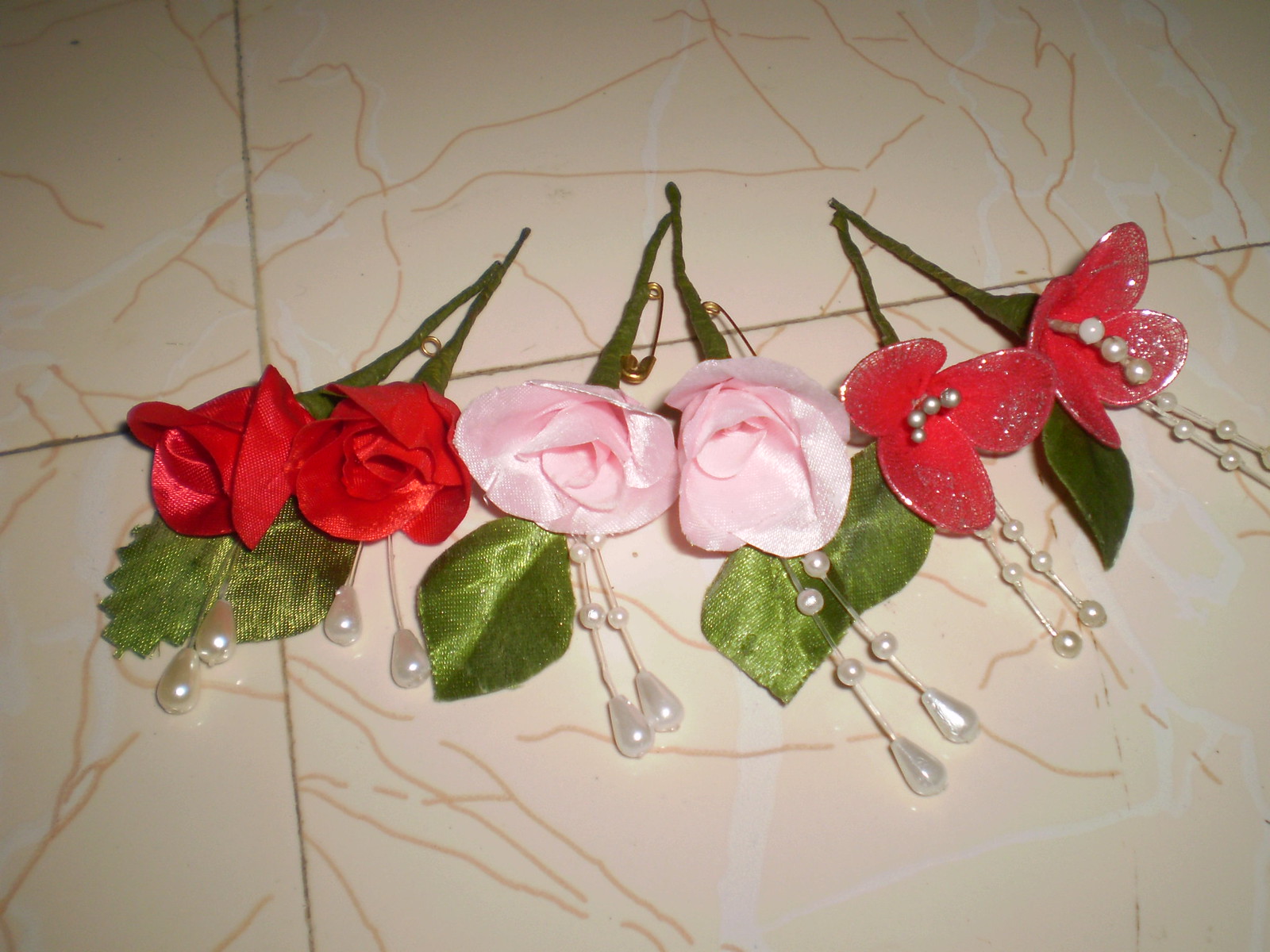This image features three silk flower boutonnieres, arranged side by side with their blossoms facing downward toward the viewer on a tan marble or formica surface. Each boutonniere showcases a different flower style meticulously crafted from a shiny silk or satin material, giving them a delicate, homemade appearance. 

The first boutonniere on the left consists of two red roses with a single leaf behind them and dual strands ending in pearls emanating from each bloom. In the center is the second boutonniere, made of two light pink roses mirroring the same elegant design as the red roses. The final boutonniere on the right displays a red poppy flower with a darker green leaf backdrop. This poppy embellished with clusters of four pearls embedded in the center and an additional pearl-tipped strand sprouting from the back. 

Each boutonniere has a wrapped green stem and a safety pin attached for fastening, emphasizing their decorative yet practical design. The arrangement is artfully displayed, capturing the intricate details of the woven petals and the glossy sheen from the light source above.